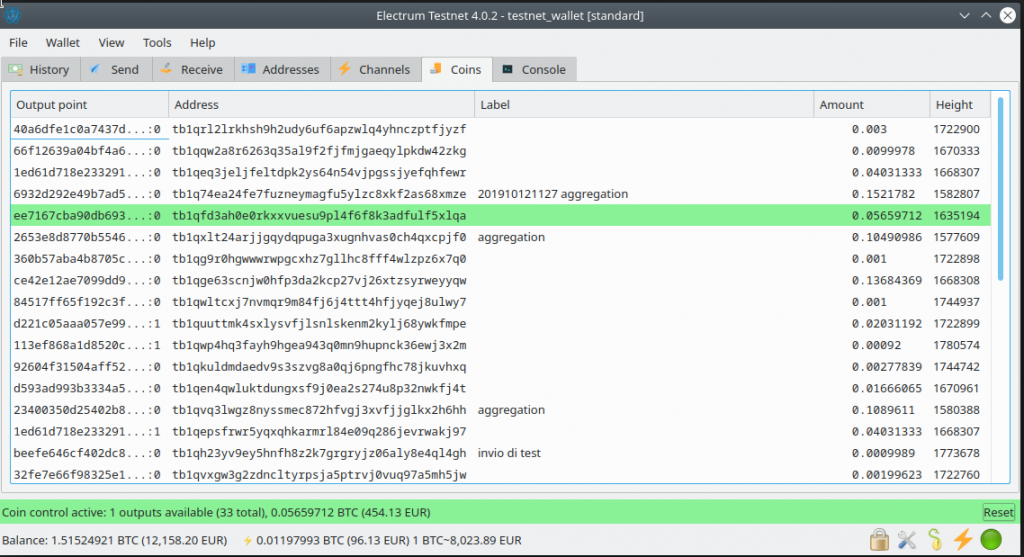The image is a detailed screenshot of an application, likely on a Windows or Linux computer, showcasing the Electrum Testnet 4.0.2 Testnet Wallet Standard. The interface is fully visible, taking up the entire image, and features a gray bar at the top with a series of drop-down menu options labeled File, Wallet, View, Tools, and Help. Below this, there are several tabs, including History, Send, Receive, Addresses, Channels, Coins, and Console, with the Coins tab currently selected. 

The screen displays a structured layout with clearly visible sections and columns labeled Outpoint Point, Address, Label, Amount, and Height. Highlighted in lime green text are an address and some numerical details. The bottom section also features lime green text, indicating a balance of 454.13 euros, equivalent to 0.05659712 BTC. The color scheme is comprised of gray, white, blue, orange, green, light blue, and yellow, which are well utilized to make the interface easy to read and navigate. 

This screenshot provides a comprehensive view of a crypto wallet in test mode, displaying various addresses, transaction details, and overall balance clearly.